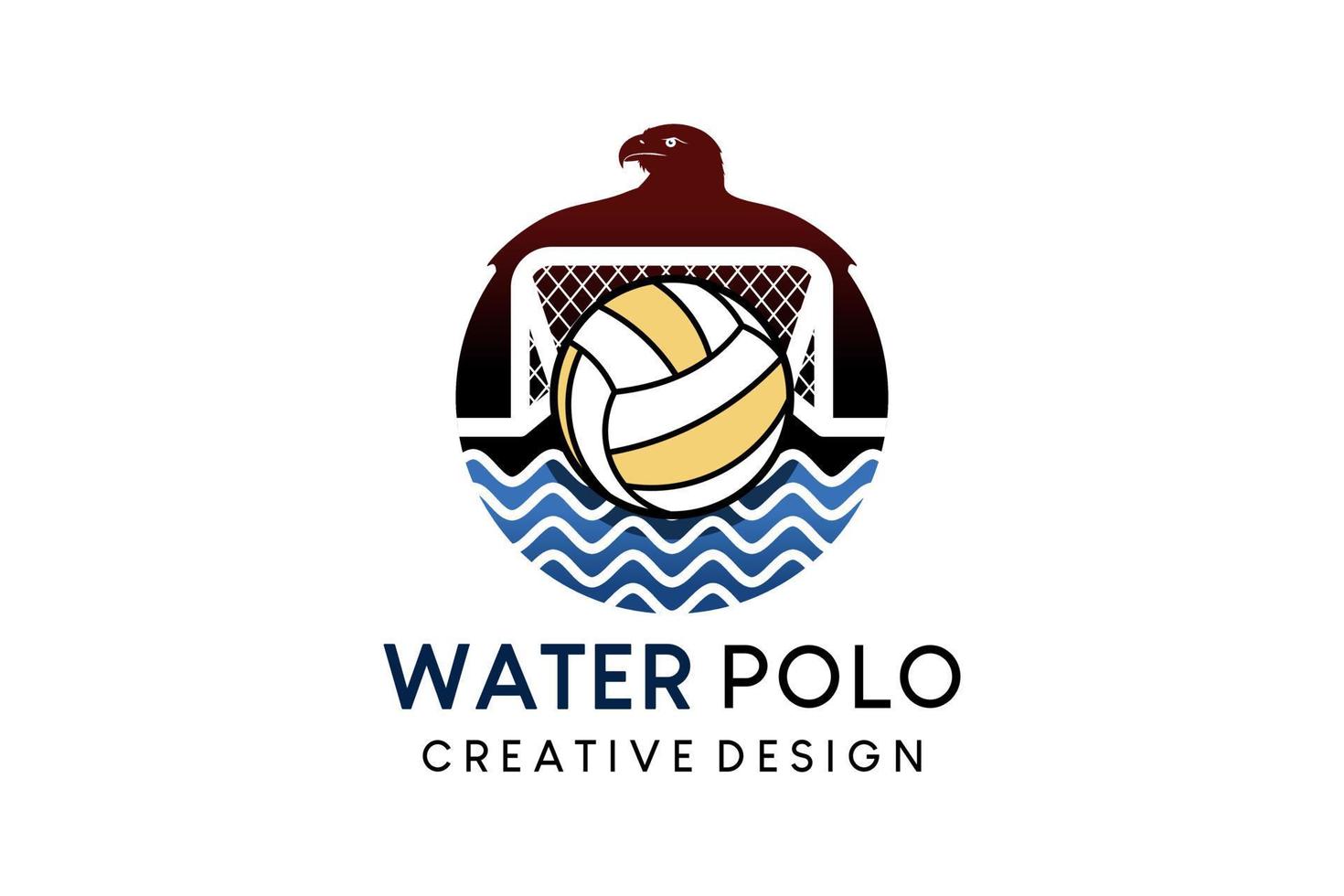This detailed color logo, set against a white background, prominently features the head of a maroon eagle at the top, with its fierce white eye and black pupil, beak pointed to the left. The eagle's wings create a rounded shape, encompassing a water polo net depicted in white against a black background. Positioned centrally over the net is a water polo ball, segmented in white and gold with black outlines. Beneath the net and the ball are stylized blue waves highlighted with white squiggles, symbolizing water. This is all encompassed in a circular design. Below this intricate logo, bold black text reads "Water Polo," with smaller text underneath stating "creative design."